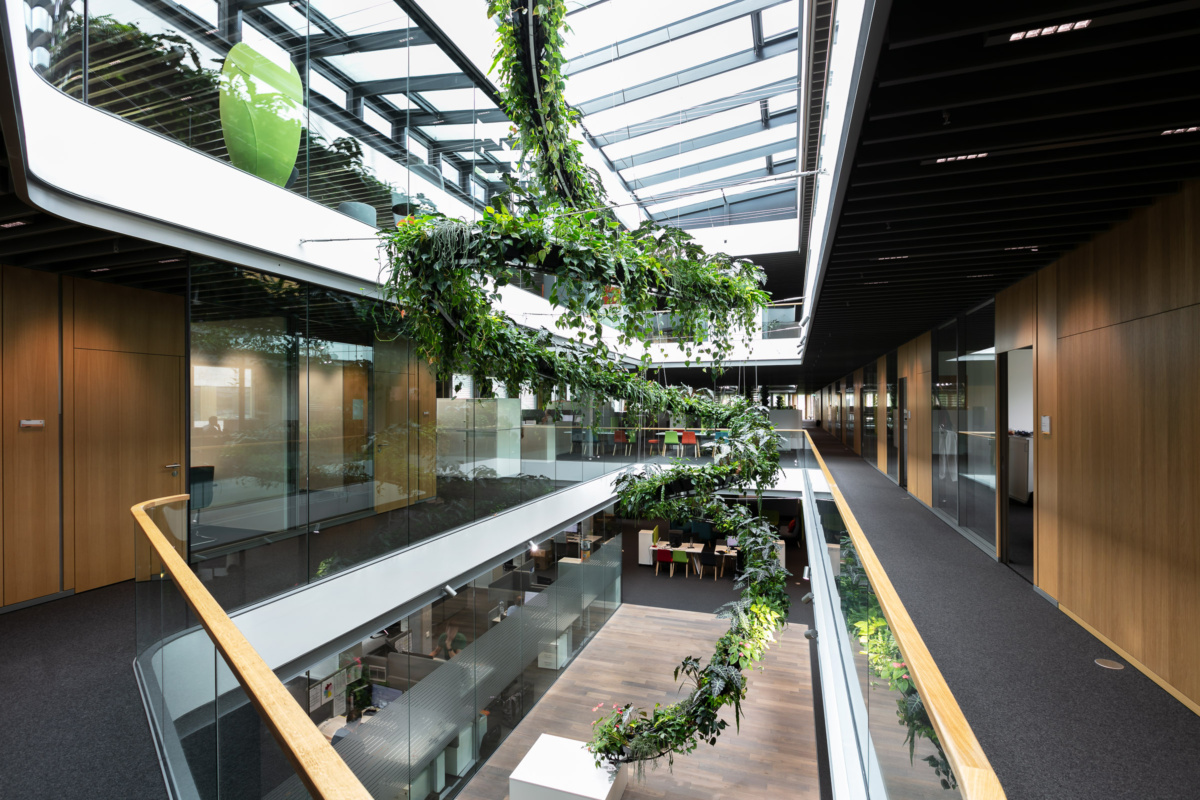The image showcases the interior of an office building with at least three levels. The primary focus is on an expansive, open central area visible from the perspective of the second floor. Above this open space is a large skylight, providing ample natural light. From the ceiling, a decorative tendril or ivy plant structure corkscrews down to the floor below. The main section where the photo is taken features dark gray carpet, which contrasts against the backdrop of brown wood paneling and floor-to-ceiling glass windows of numerous small offices. The first floor beneath has a hardwood finish and appears to be a meeting area with a large table and workspace cubicles to the left. Hallways on both sides of this central atrium are lined with office doors, offering a clear look into the bustling workspace below. The overall architectural design evokes a blend of modern utility and natural elements, contributing to a dynamic and airy office environment.